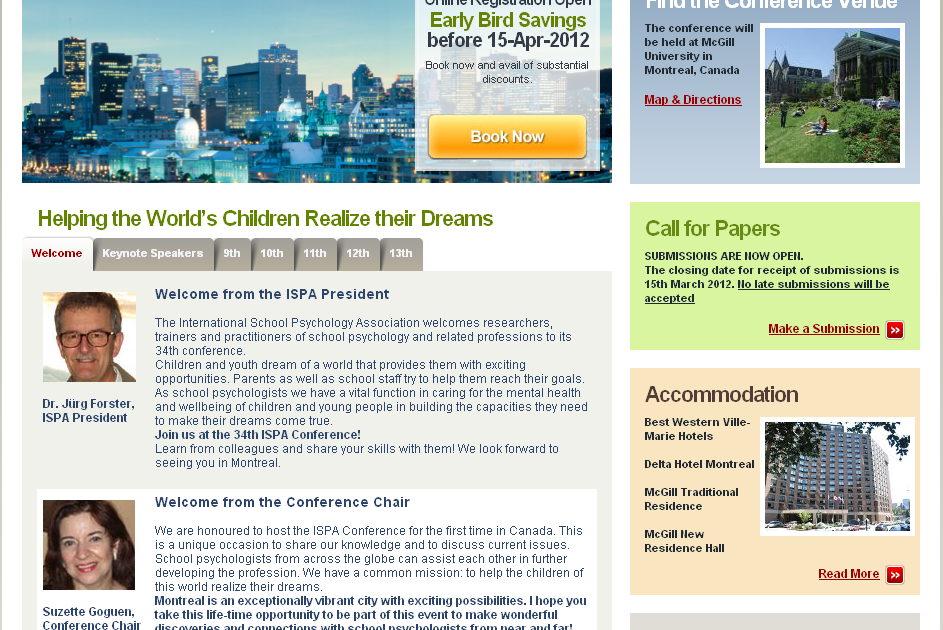**ISPA 34th Conference Announcement - Key Highlights**

The image appears to be an announcement for the 34th International Psychology Association (ISPA) Conference, featuring a variety of notable elements and details. 

At the top of the document, there's a highlighted section that mentions "Early Bird Savings Before April 15, 2012," indicating a promotional period for reduced registration fees. Next to this, a "Book Now" button is prominently displayed.

To the right, several important components regarding the conference are listed:
1. **Conference Location**: The event is scheduled to take place at McGill University. A clickable link provides a map and detailed directions.
2. **Call for Papers**: Submissions are currently open, with the option to submit proposals in PDF format.
3. **Accommodation**: Various lodging options are mentioned, including Best Western and some residence halls.

On the left side, there's a welcoming message from Dr. Jurg Forster, ISPA President. His introduction gives a brief overview of his background and his association with ISPA. He extends an invitation to researchers, trainers, practitioners, and related professionals to attend the conference.

Additionally, the message includes a note from Suzette Gorkson, the Conference Chair, who expresses her honor in hosting the ISPA conference in Canada for the first time.

There is also a navigation menu with several tabs, including:
1. **Welcome**: Featuring messages from Dr. Jurg Forster and Suzette Gorkson.
2. **Keynote Speakers**: Information about the keynote speakers scheduled for the event.
3. **Various Dates**: Tabs marked with "9th," "10th," "11th," "12th," and "13th," likely corresponding to the dates of the conference or specific sessions.

This descriptive breakdown provides a comprehensive view of the conference details available within the image.